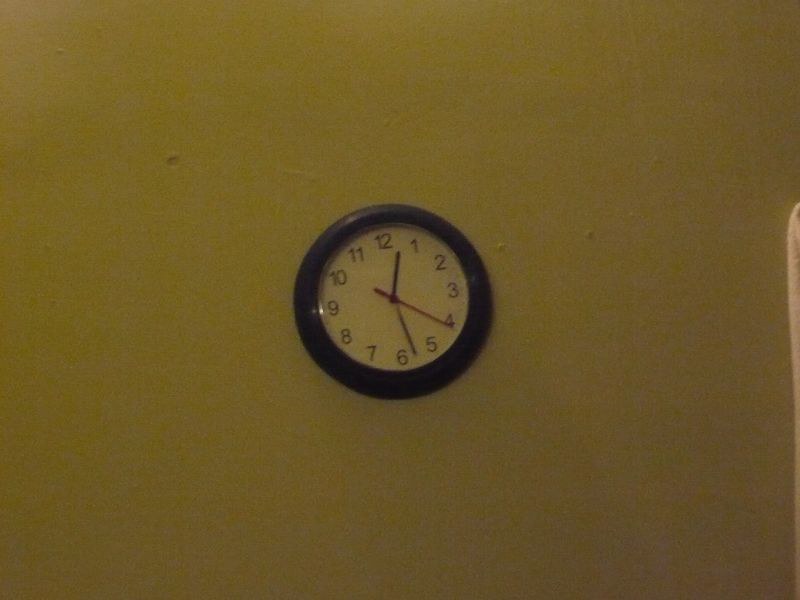This color photograph captures a slightly skewed clock mounted on a mustard-colored wall. The clock, which is tilting slightly to the left, has a thick, curved border that appears to be dark in color, possibly black or dark wood. Its face is white, encircled by a sequence of black numbers from 1 to 12. The clock's hour hand sits between the 12 and the 1, while the minute hand points between the 6 and the 5, indicating a time around 12:28. Just past the number 4 is a slender red second hand. A small detail, possibly the edge of a pink shirt, intrudes slightly from the right side of the image. The overall effect of the photograph is slightly soft and the picture is rectangular in shape.